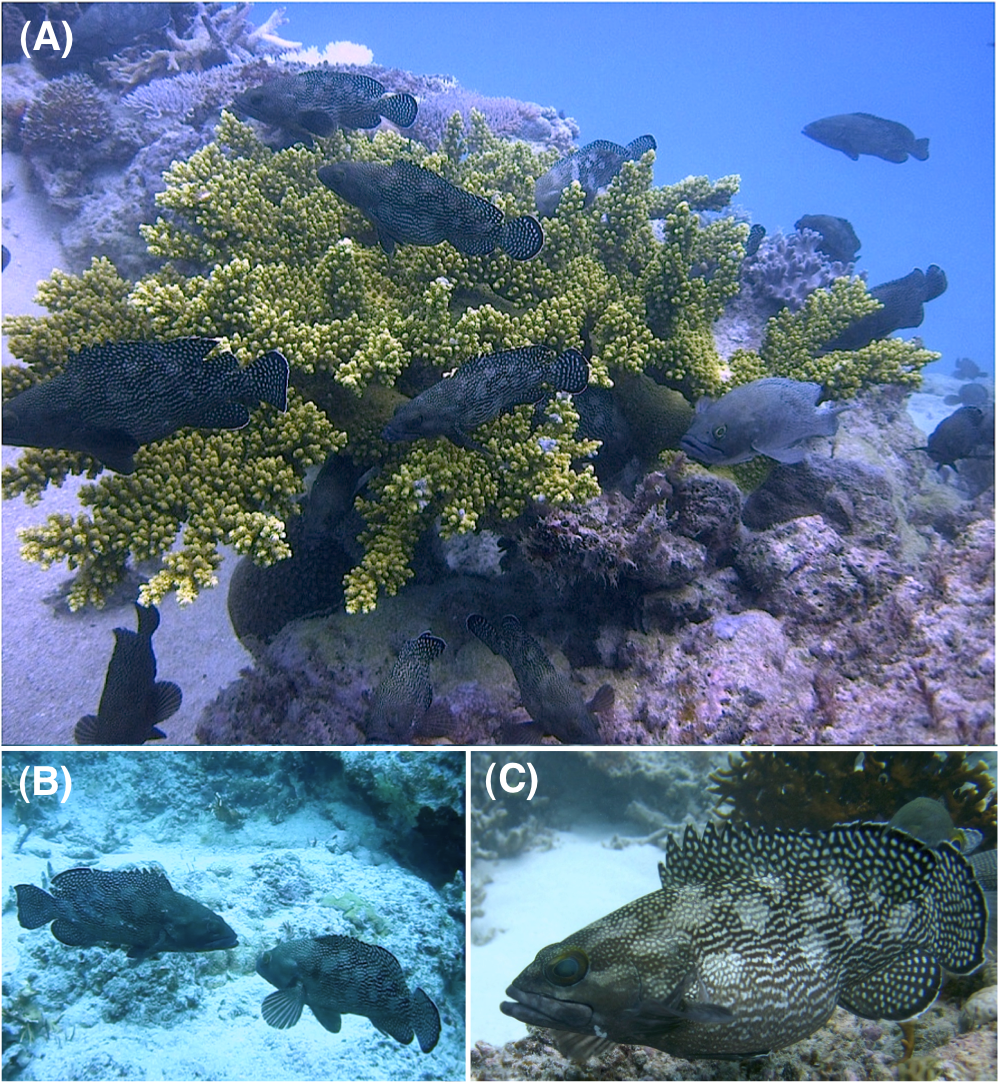The collage image showcases three underwater scenes, labelled A, B, and C. Image A, the largest at the top, depicts a vibrant underwater environment with clear, blue water. In the middle of the frame, there's a cluster of green, textured plant life attached to a rocky, brown seabed. Surrounding the plants are several dark grey fish, their scales subtly reflecting shades of purple under the light. The shadowy depths of the water add a sense of depth and clarity to the scene.

Image B, located at the bottom left, features two dark grey fish facing each other against a bluish background. The fish have rounded, short tails and streamlined bodies, with elongated fronts. There are hints of a white encrusting area blending into the darker backdrop, adding contrast to the scene.

Image C, in the bottom right, focuses on a singular, larger grey fish with a bulbous midsection. This fish is distinctively detailed with intricate round markings and black and white dotted patterns. The background here is greyish, but there's a splash of green plant life faintly visible. The fish's ornamental appearance, combined with the textured seabed it glides over, completes the marine tableau, teeming with underwater life.